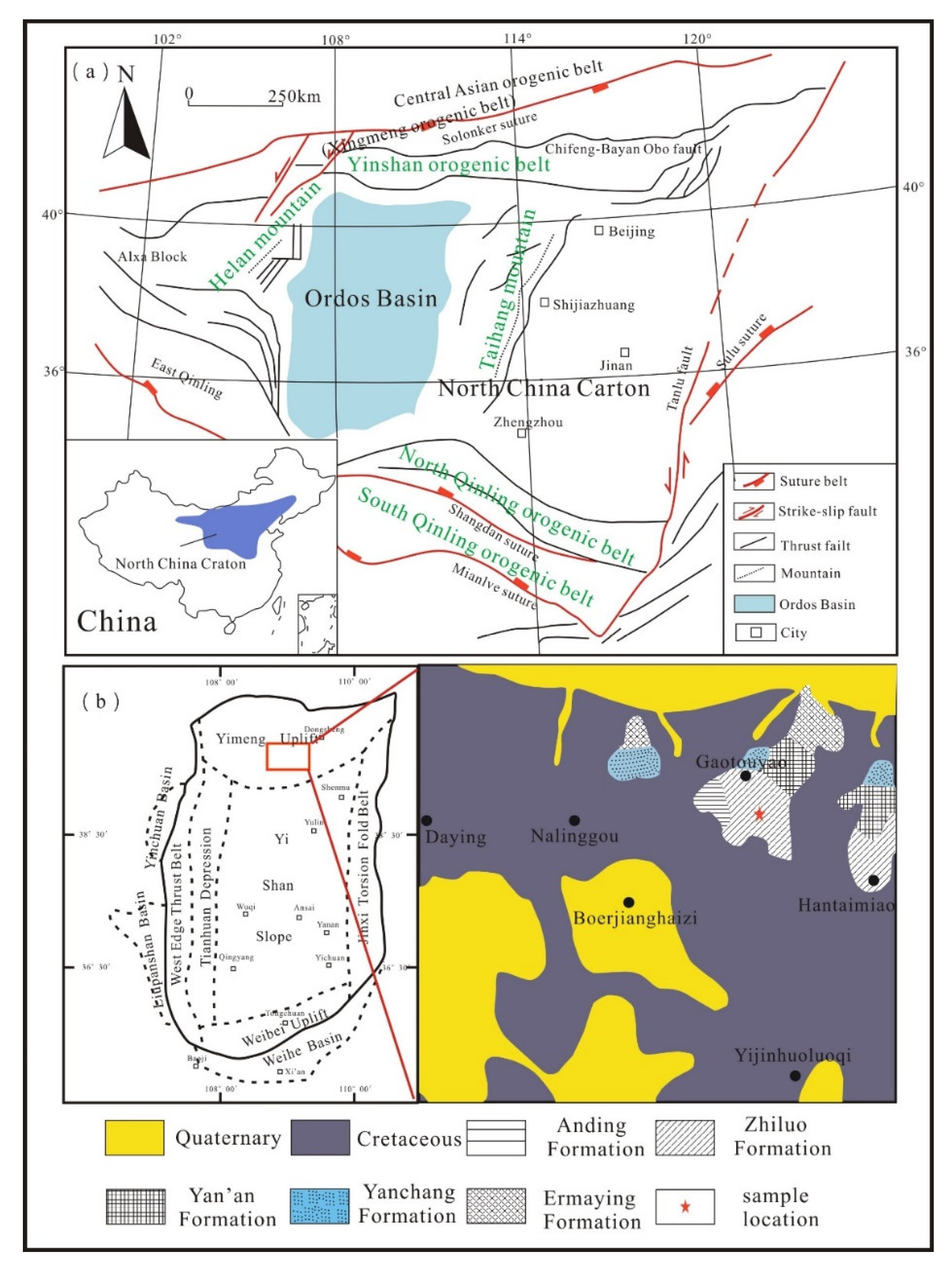This image depicts a detailed set of maps showing different geological and geographical features in China, focusing on the North China Carton and Ordos Basin. The central and largest of these maps shows an irregular blue shape labeled Ordos Basin, surrounded by various red and black lines denoting geological structures such as Suture Belt, Strike Slip Fault, Thrust Fault, Mountain, and City. Latitude and longitude lines are present, along with a north-pointing compass.

Additionally, adjacent maps provide focused insets of specific areas: the bottom left map illustrates a circular region known as the West Edge Thrust Belt, marked by distinctive red straight lines and black dotted lines. The bottom right map, colored dark purple and yellow with black and white plaid and stripes, includes names of locations such as Daying, Nilingu, Gastayao, Bo, Gazi, Jin, Hu, and Luozhi. Both of these smaller maps have corresponding keys in the bottom sections that clarify the different colors and symbols used to represent the various geological and geographical elements.